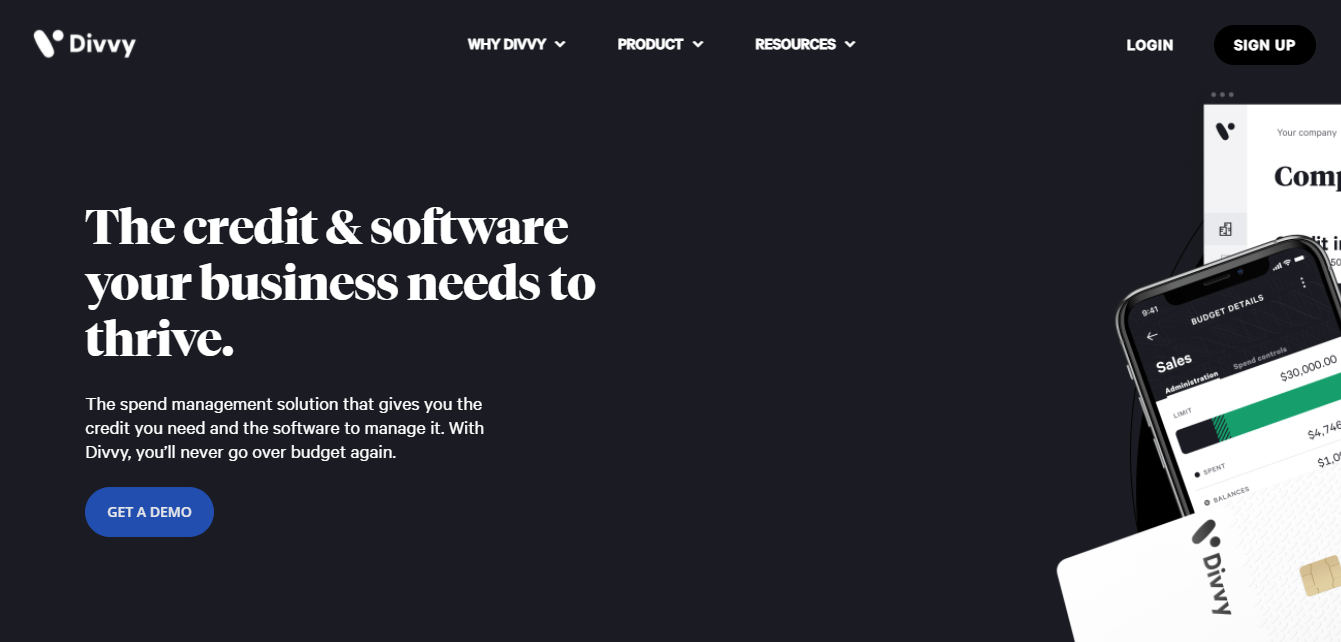**Caption:**

This is a detailed advertisement featured on a website with a dark gray background. The design is a long horizontal rectangle. In the top left corner, a large, bold "V" is prominently displayed, next to which the brand name "Divvy" (spelled D-I-V-V-Y) appears. Centered at the top, there are three dropdown menu items labeled: "Why Divvy," "Product," and "Resources," each accompanied by a downward arrow. The top right corner houses the "Login" button and a "Sign Up" button contained within a black oval.

The main text on the left side reads: "The credit and software your business needs to thrive." Beneath this, in smaller font, the tagline states: "The spend management solution that gives you the credit you need and the software to manage it. With Divvy, you'll never go over budget again." Below this, a blue oval button labeled "Get a Demo" invites users to take action.

On the right edge of the advertisement, a smartphone is depicted. A credit card with a chip, branded with the Divvy logo, lies sideways across the bottom of the device, partially covering a sheet of paper. The image collectively highlights Divvy's spend management and business credit solutions.